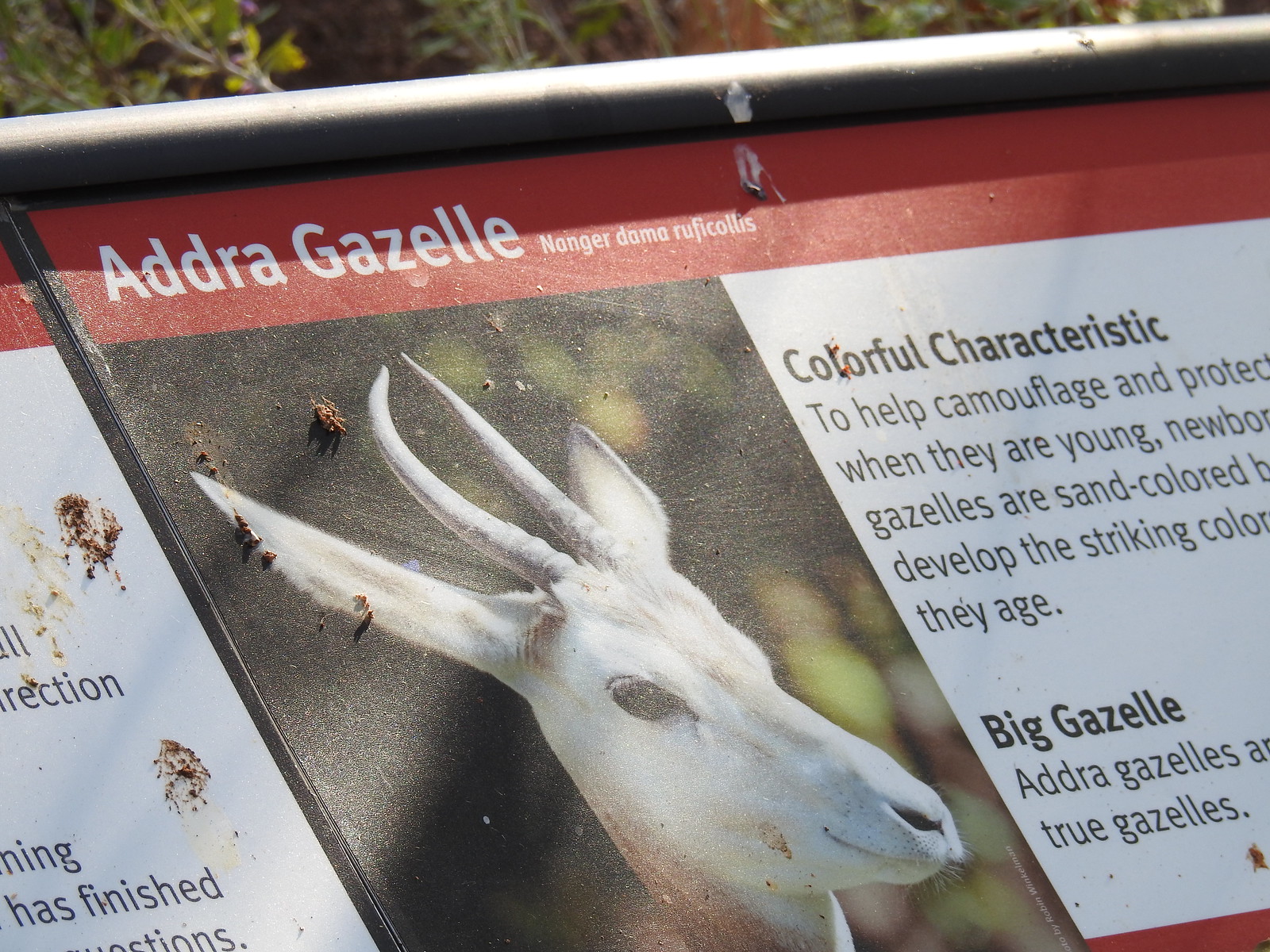The image depicts an informational plaque typically found in a zoo, placed near an animal enclosure. The plaque, encased in a black metal frame, features a photograph and description of an Adra Gazelle. At the top, a red banner with white text prominently labels the animal as "Adra Gazelle." The accompanying text, though partially obscured, mentions the gazelle's "colorful characteristic to help camouflage and protect when they are young." It further explains that newborn gazelles are sand-colored before developing their distinctive, striking coloration as they age. The plaque continues with information on the size of the gazelle, starting with "Big gazelle, Adra gazelles..." but the subsequent text is unreadable. To the left of the text is an image of the gazelle, notable for its white face and two prominent horns. The plaque is slightly marred by bird feces, indicating it is situated outdoors, with some green foliage visible in the background.